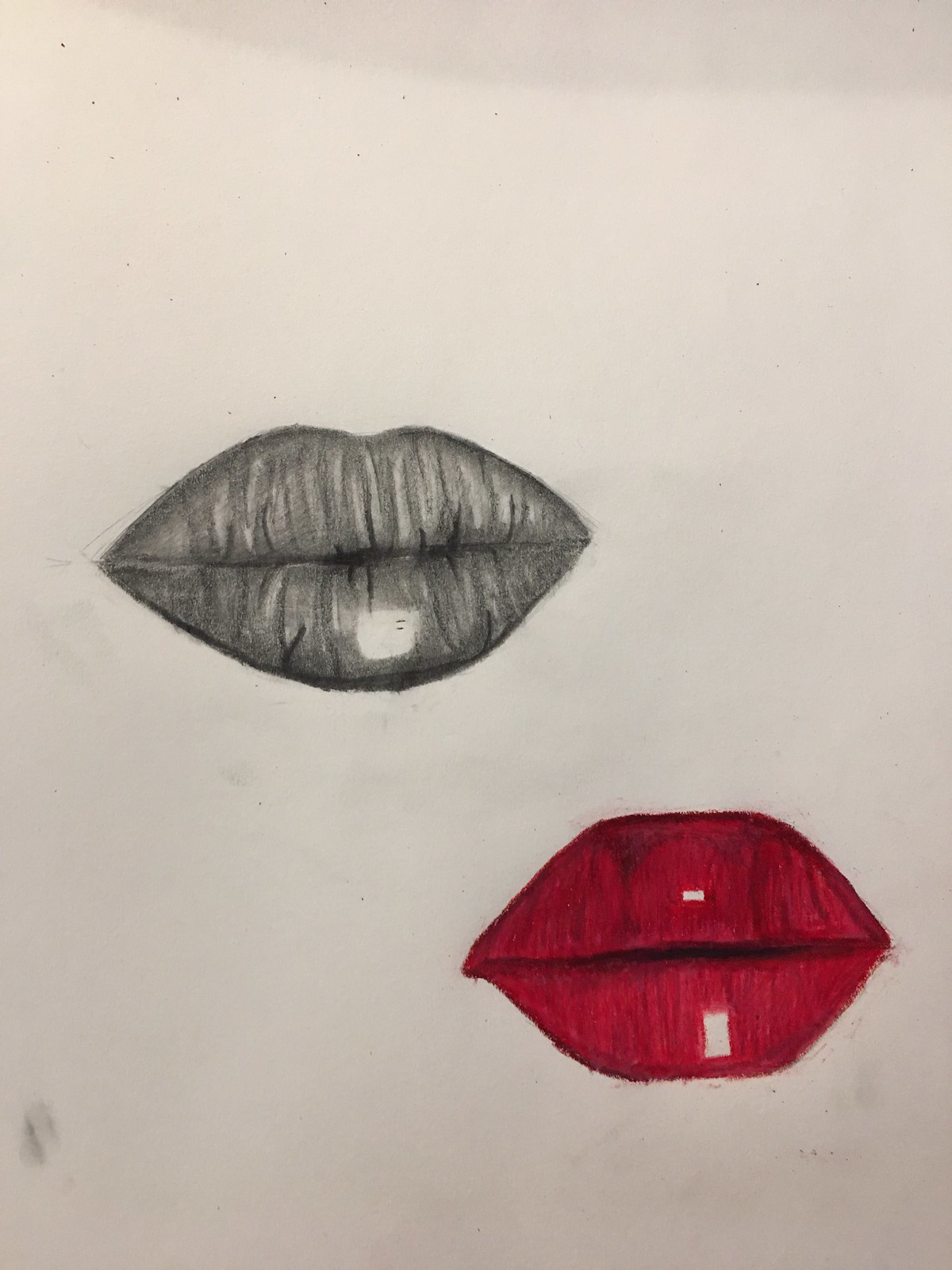On a white background featuring pencil sketches, there is a highly detailed illustration focused on the left side and the bottom-right corner. To the left, a prominently highlighted and carefully drawn lip stands out, accompanied by a distinct white reflection at its bottom, giving it a glossy appearance. The background around this lip area is mostly grayed out, framed by a darker black border that enhances the contrast.

In the bottom-right corner, another set of lips are depicted, with delicate shading and intricate detail. These lips have a subtle whiteness at the mouth, progressing to darker tones towards the center, which adds depth to the image. The lips are predominantly light red with the edges shaded in a darker red, creating a striking visual contrast that captures the viewer's attention. The entire composition is defined by light and shadow, bringing a realistic touch to the sketched lips.